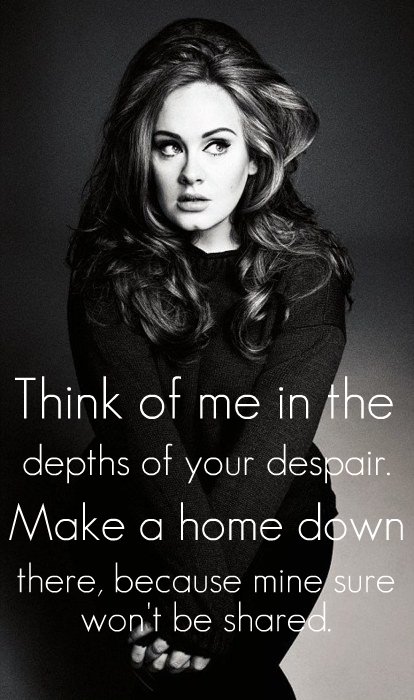This black-and-white image features the iconic singer Adele prominently in the center, extending almost from the top to the bottom of the frame. The background transitions from a darker black or gray at the top to a lighter gray at the bottom, creating a gradient effect. Adele, with her long, curly dark hair, is depicted in a thoughtful pose, looking off to the side while her hands rest on her knees, suggesting she might be crouching. She is dressed in a long-sleeved, dark gray or black sweater and dark pants. Across the lower third of the image, in bold white letters, are lyrics from one of her songs: "Think of me in the depths of your despair. Make a home down there because mine sure won't be shared." The image captures a somber yet powerful mood, reflective of Adele’s emotive music style.